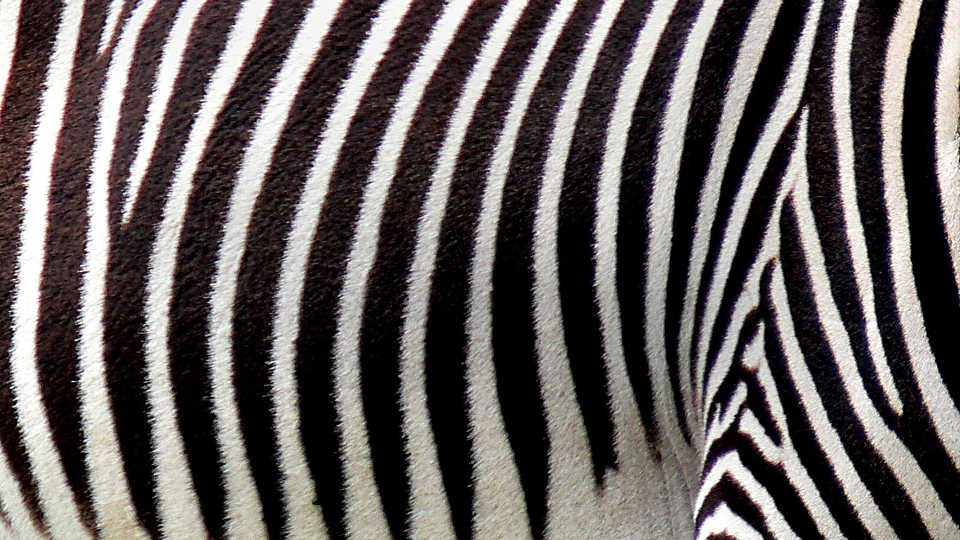This close-up image captures the side view of a mature zebra, accentuating its distinctive black and white vertical stripes. The animal's fur appears unexpectedly fluffy, reminiscent of mohair, creating a textured and vivid contrast between the intense dark black and striking raw white stripes. The shot likely captures the zebra from the front, hinting at a leg or front haunch emerging from the lower right corner, where the stripes narrow and form a V-shape toward the belly. The detailed view highlights the mesmerizing pattern and fur texture, although the zebra's head and tail are out of frame.